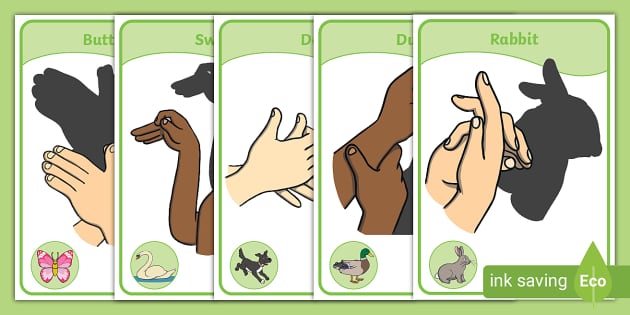This image shows five trading card-shaped illustrations, each depicting a different animal through hand shadow puppets. The cards are partially overlapping, but the one featuring a rabbit is fully visible. Each card has a consistent design: a green banner at the top with the animal's name in green text, an illustration of hands forming a shape to create the animal's shadow, and in the bottom left corner, the animal itself depicted in a green circle. The cards have white outlines accented by a smaller green outline with rounded corners.

The animals featured are a butterfly with pink wings and a yellow body, a swan depicted on a bed of water, a black and white dog, a duck with a green head and yellow beak, and a gray rabbit with pink ears and a white tail. The cards illustrate the hand positions necessary to create each animal's shadow. Additionally, there is text in white with an ECO logo and a teardrop icon at the bottom right, promoting ink-saving features.